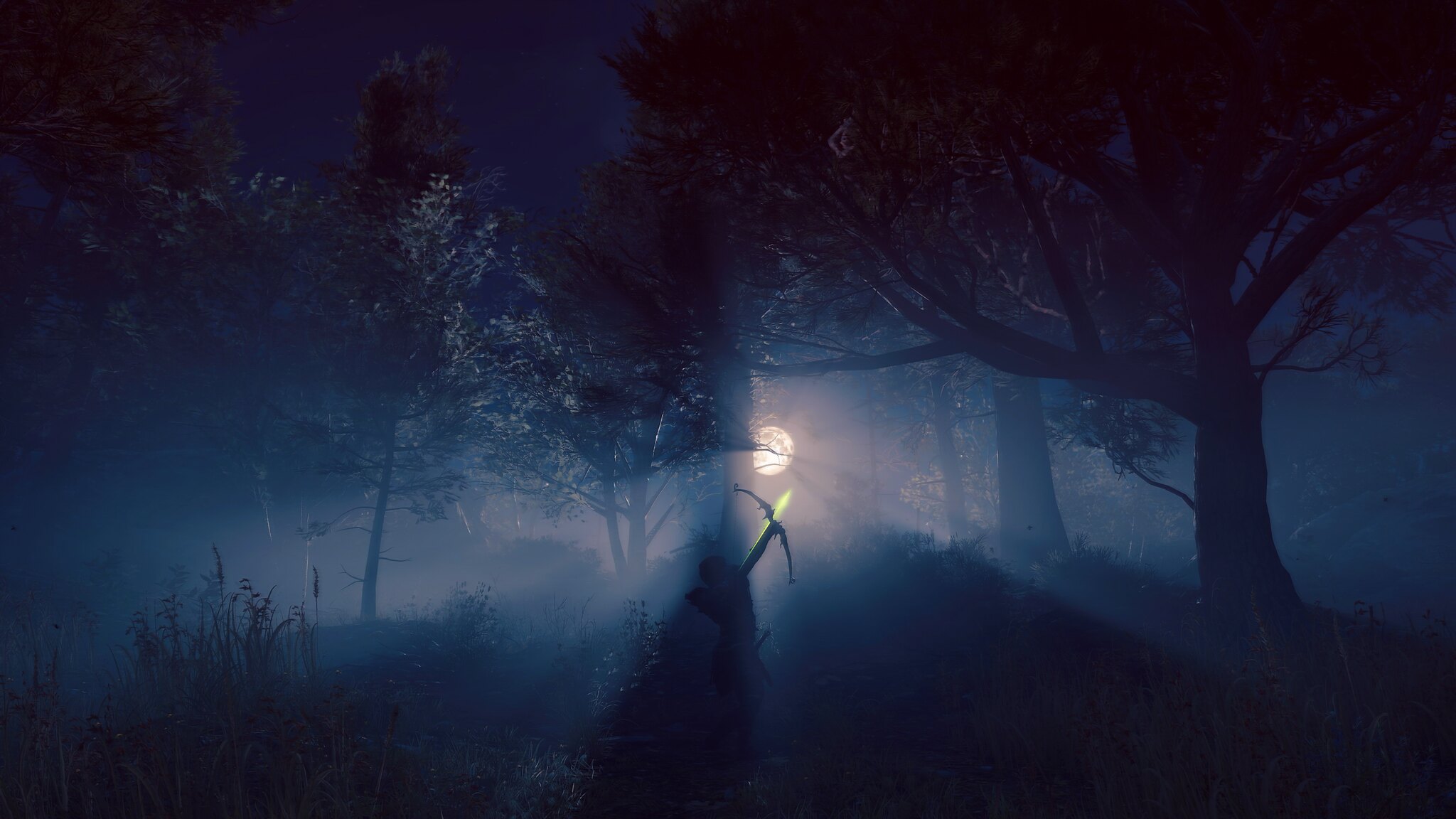In the image, we observe a mystical nighttime forest bathed in the dim yet luminescent glow of a full moon, casting a white-grayish hue across the scene. The forest is dense with vegetation; tall grasses occupy the bottom left corner while a mix of thick, big-trunked trees and slender, smaller trees frame both the left and right sides. The moonlight beams through the foliage, creating an ethereal atmosphere accentuated by a thin layer of fog drifting through the center. Silhouetted against this moonlit backdrop is a figure standing in the center, mostly cloaked in shadow. The person, dressed in black, is holding a black crossbow with a flaming green, energy-like arrow. The serene yet eerie setting, featuring detailed silhouettes of tree branches and leaves, adds to the otherworldly ambiance of the forest.